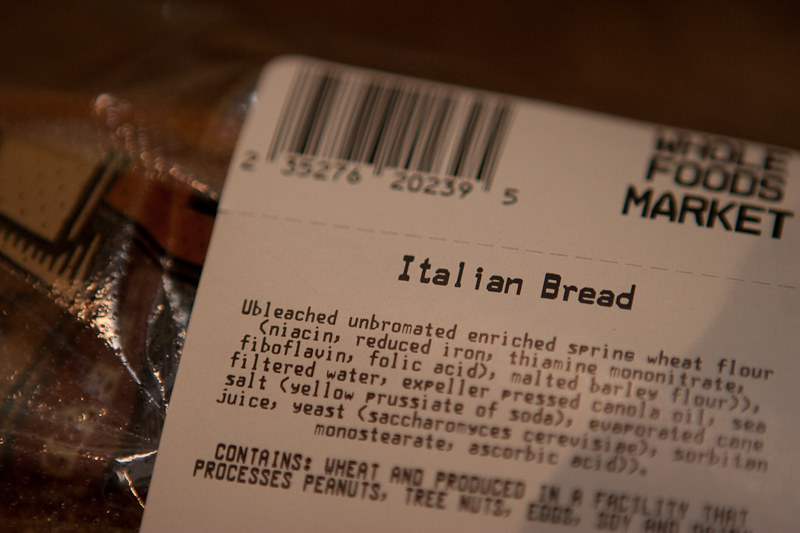The image features a labeled plastic bag containing Italian bread from Whole Foods Market. The label, positioned prominently on the bag, details the following product information: "Whole Foods Market" and a barcode to the left. The bread, described as Italian, includes ingredients such as unbleached, unbromated, enriched brine, wheat flour, niacin, reduced iron, thiamine mononitrate, riboflavin, folic acid, malted barley flour, filtered water, expeller-pressed canola oil, sea salt, yellow prussiate of soda, evaporated cane juice, saccharomyces cerevisiae, sorbitan monostearate, and ascorbic acid. It also notes that the product contains wheat and is produced in a facility that processes peanuts, tree nuts, eggs, and soy. The image shows this label in clear focus on the upper middle right, while the surrounding plastic wrap appears both at the top and bottom left. Hints of beige, brown, and orange colors are visible, though it's unclear if they are part of the bag or background. The top portion and bottom right corner of the image are relatively fuzzy, albeit still discernible.